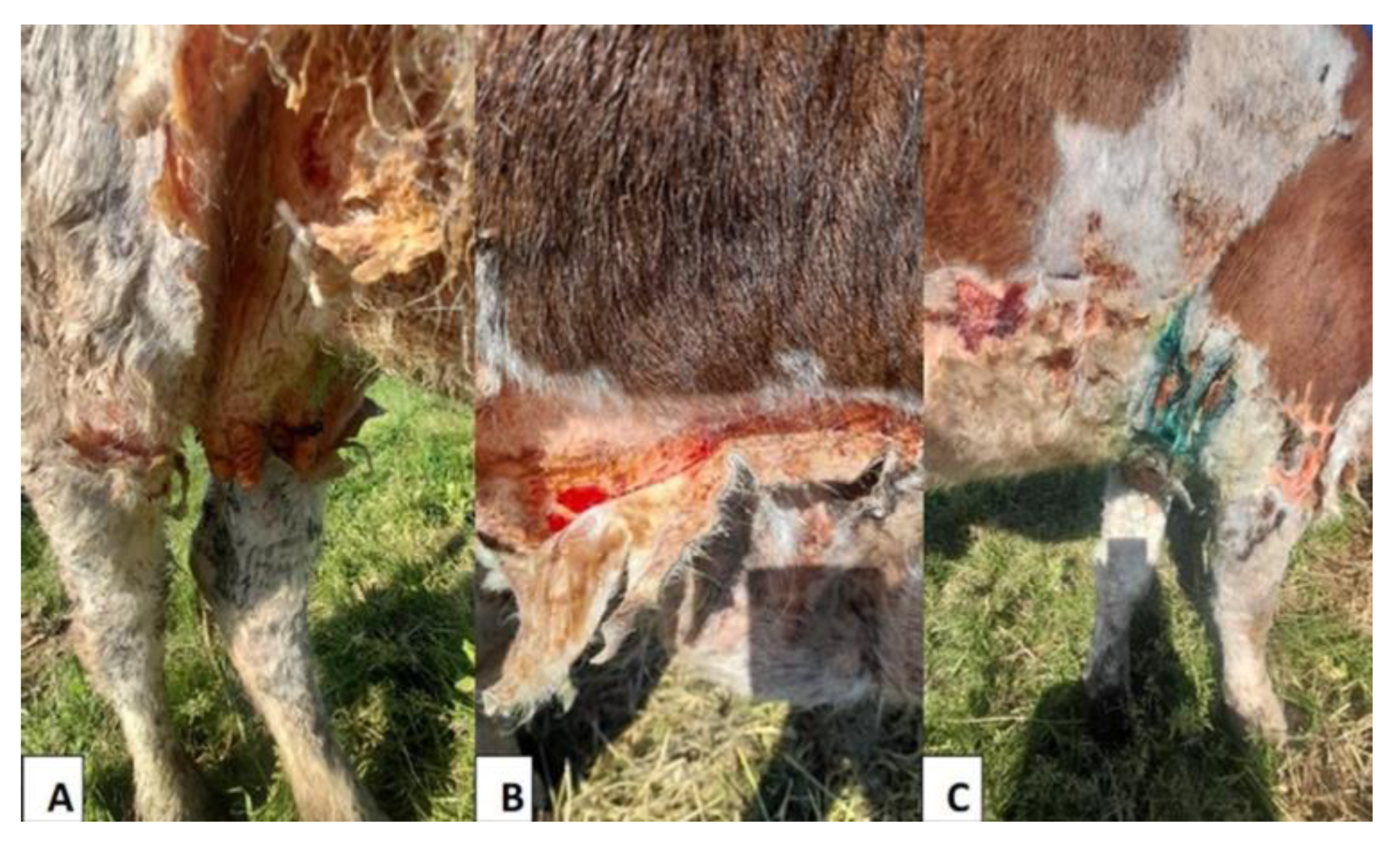The photograph is divided into three labeled sections: A, B, and C. Each section showcases different views of a furry, four-legged animal, possibly a cow or sheep, standing on greenish-yellow grass. Section A highlights the animal's off-white to grayish fur with visible reddish-orange lacerations and wounds, particularly around its belly and legs. Section B focuses on the animal's abdomen, displaying severe injuries with torn hide, exposed flesh, and some blood, suggesting an attack or an accident. The brown fur in this section looks particularly ragged. Section C shows an attempt to patch up the animal's injuries, with some mended fur and efforts at treating the wounds. Collectively, the image portrays the distressing state of an injured animal with detailed depictions of the damage it has suffered and initial steps towards its recovery.